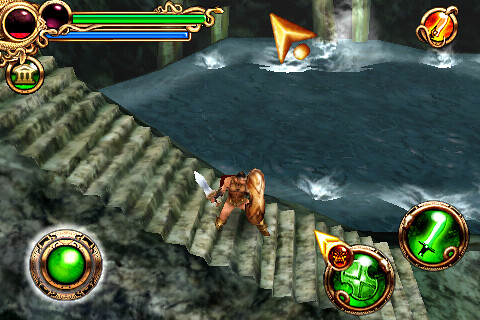This screenshot from a 3D video game features a burly warrior, possibly inspired by ancient Greek or mythological themes, descending an imposing marble staircase that diagonally bisects the image from the upper left to the lower right corner. The warrior, with an imposing build, is depicted wielding a massive sword in one hand and an equally large gold shield in the other, which nearly matches the height of his body. His face is not clearly detailed, evoking a somewhat enigmatic presence. Surrounding him is a dark, disturbed body of water, complete with splashes and ripples, hinting at recent activity. Behind him, there is possibly a waterfall feeding into this water. The game’s user interface is dense with cryptic icons and bars: the upper left corner shows likely health and mana bars in green and blue respectively, while the lower section displays various skill and ability icons in neon green with gold accents. Additionally, a prominent navigational tool featuring a large green gem is positioned at the bottom left. The presence of a large gold arrow cursor suggests some level of modernity in the game’s design, albeit with a nostalgic aesthetic.